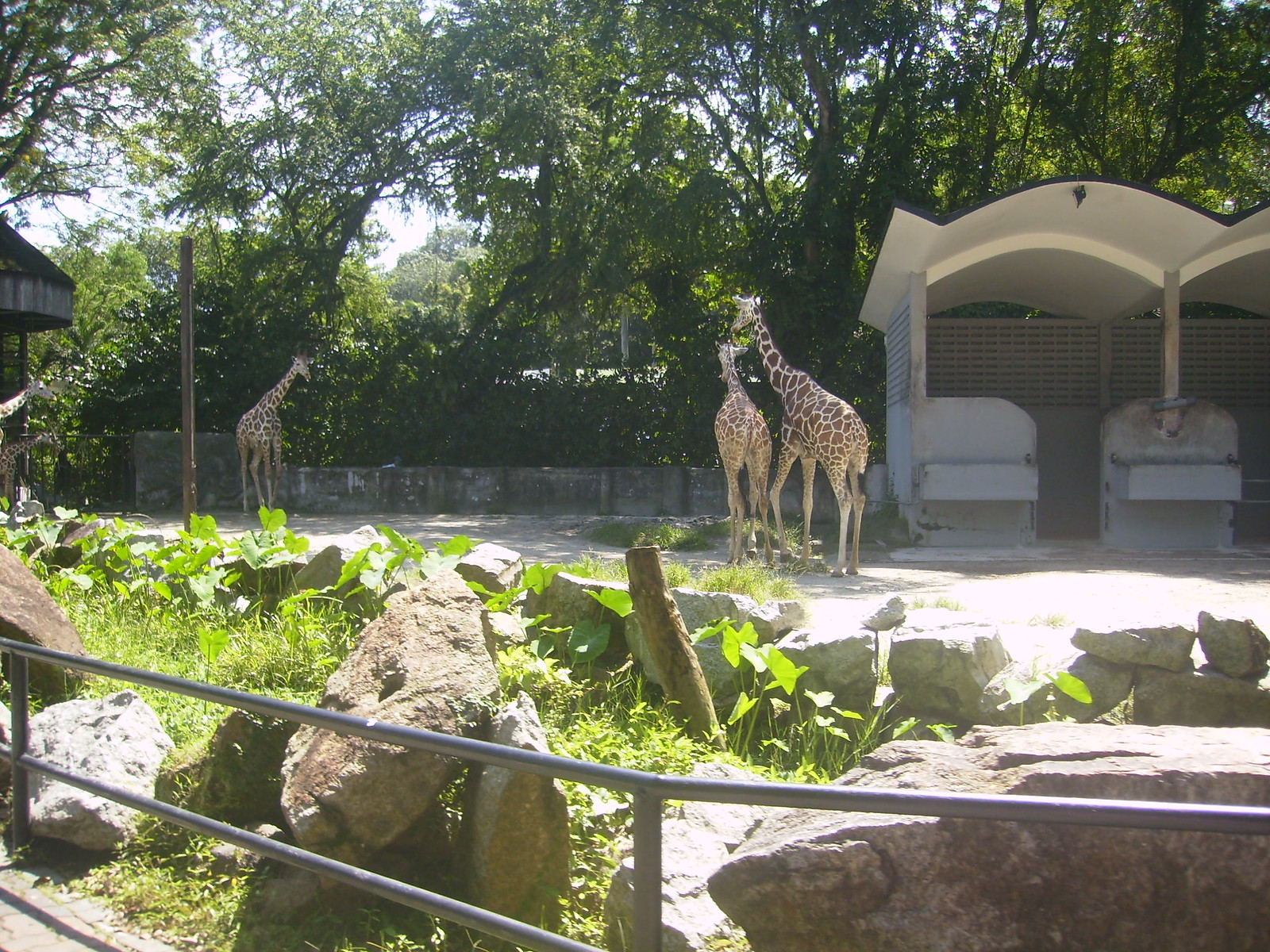The image depicts a bright, sunny day at a zoo, showcasing a detailed open-air giraffe enclosure. There are three giraffes present: two are positioned just off to the right of the center, facing away from the camera, while the third is situated further back on the left, slightly facing the camera and standing next to a wooden pole. The ground within the enclosure appears to be a mix of light dirt and concrete, dotted with tufts of grass.

In the foreground, a metal railing runs across the bottom of the photo, separating the viewer from the giraffe habitat. Behind this railing, the area features several large rocks and patches of greenery, followed by a small brick wall made from white granite that stands about three feet tall. This brick wall extends along the enclosure, creating a six-foot barrier from the giraffes.

To the right of the enclosure is a metal structure with a curved roof and latticework walls, likely serving as a covered feeding station for the giraffes. Further back, a brick wall runs along the back of the enclosure, with numerous trees rising behind it, enhancing the scene's natural ambiance. The overall scene is slightly overexposed but provides a clear and vibrant depiction of the giraffes and their habitat.